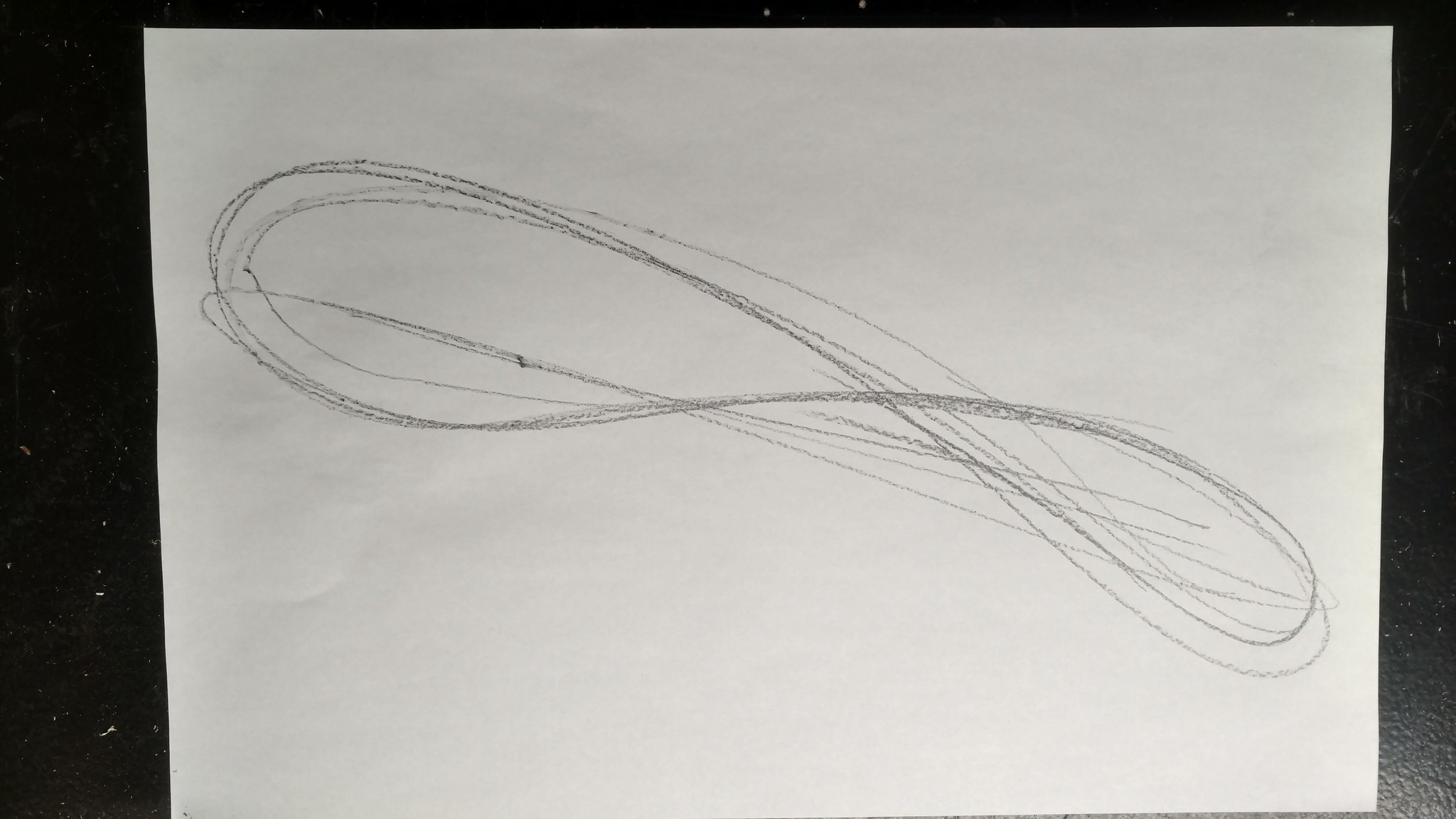A white sheet of paper lies prominently against a subtly textured gray background, which initially appears black. On the left edge, faint glimmers of light reveal the presence of an unseen object. The background, though largely dark, has discernible gray patches, particularly on the bottom right corner. Dominating the sheet of paper is a large, intricately sketched infinity symbol, positioned slightly askew, running from approximately the 10 o'clock to the 4 o'clock positions, reminiscent of elongated paddles. The infinity sign is composed of multiple pencil strokes, ranging from light to dark, indicating repeated attempts to perfect its form. Tiny dots punctuate the center of the symbol, marking the starting and stopping points of the sketches. The sketch appears unfinished, with many light lines suggesting the artist’s intent to later solidify and refine the design.